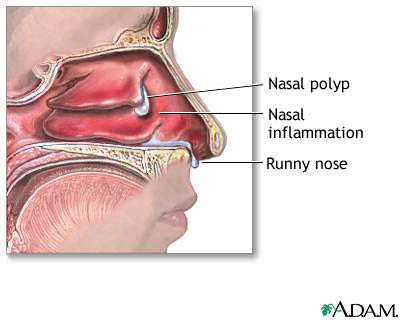This detailed medical illustration, sourced from ADAM, presents a cutaway profile of a human face, meticulously exposing the internal anatomy of the nose and sinuses. The diagram highlights various diagnostic features, such as nasal polyps, depicted as small white bubbles within the nasal cavity. It also illustrates areas of nasal inflammation, shown in red, and labels a runny nose with white fluid dripping from the nostril. The image omits the eyes but clearly displays the external lips and tongue, maintaining the typical style of medical textbook illustrations. This comprehensive breakdown provides a clear visualization of the conditions contributing to a runny nose, aiding in both diagnosis and understanding.